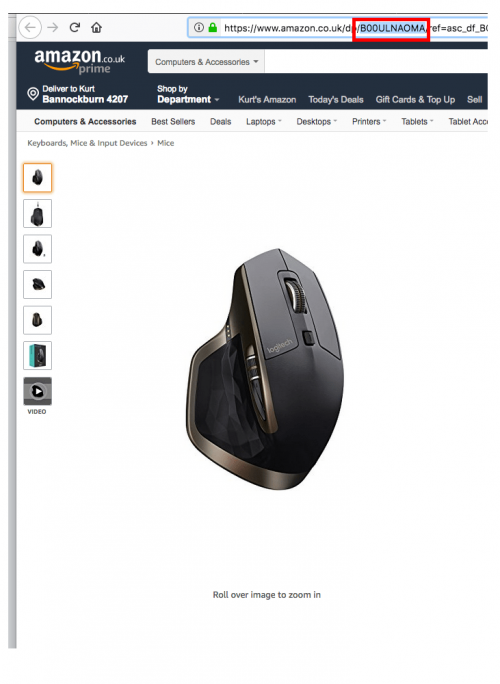The captured image from an Amazon site on a desktop computer prominently displays the left side of the screen. At the top, the address bar is visible, featuring a green padlock followed by the URL "https://www.amazon.co.uk". Directly beneath, a black header bar spans the width of the screen, adorned with the amazon.co.uk Prime logo on the left. Below this logo, several navigation options are clearly visible, including "Shop by Department," "Kurtz Amazon," "Today's Deals," "Gift Cards," and "Top Up".

The screen content primarily focuses on an image of a sleek, black computer mouse presented for sale. This detailed view offers a snapshot of the browsing experience on Amazon's UK website, highlighting both the website's structured navigation interface and the specific product being shown.